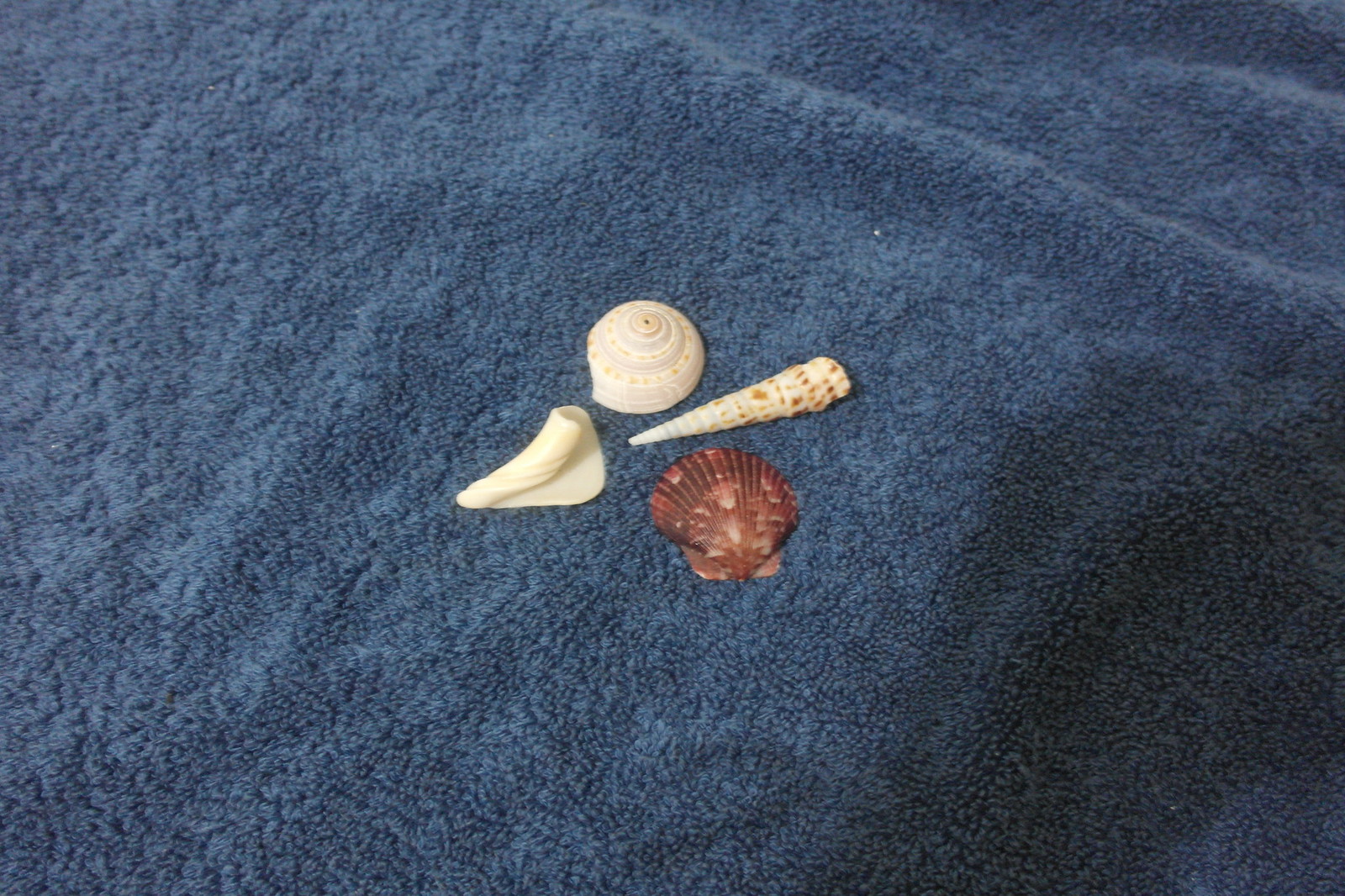The image features a top-down view of four distinct seashells laid out on a blue piece of cloth, possibly a towel that is somewhat bumpy and hastily spread over a flat surface. Centered in the photograph, these seashells form a small cluster with each showcasing unique characteristics. 

The top shell is a conical, spiral shell reminiscent of a snail or a hermit crab's home, predominantly white in color. To its right lies another conical shell, elongated like a narwhal's horn, white with orange or brown speckles. Below these, there's a classic scallop-shaped shell, dark brown with lighter cream spots, positioned with its concave side facing downward. The leftmost shell in the arrangement appears flattened and twisted, similar to a rolled cigarette or a piece of curled paper; it is completely white.

Together, these four seashells create a visually intriguing and diverse collection against the rich blue backdrop.